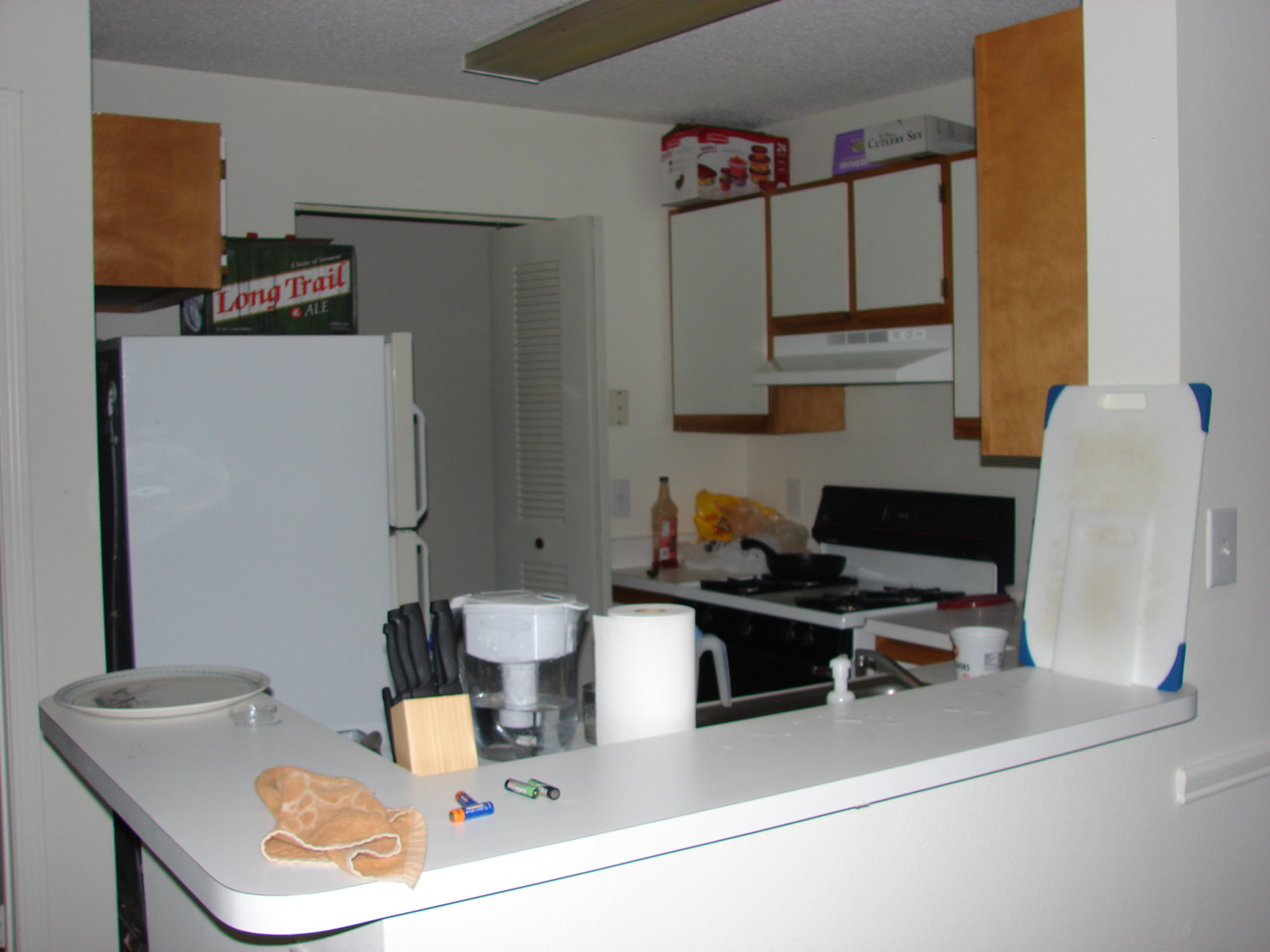This photograph captures a cozy, small kitchen viewed from an adjoining room through an open passageway. The kitchen is partially separated by an L-shaped white breakfast bar that serves as a functional countertop area. Draped casually on this breakfast bar is a loosely folded peach-colored hand towel. A set of AA batteries and a well-used white plastic cutting board with blue corner borders rest against the wall on the counter. An empty dinner plate perches on the edge of the breakfast nook side of the bar.

In the kitchen beyond the breakfast bar, a Brita water pitcher half-full with water accompanies a roll of white paper towels on the countertop. A wooden knife block holds an array of knives with black handles, their blades securely sheathed within. A metallic faucet is visible above a stainless steel sink, emphasizing the practical side of this kitchen.

Perpendicular to the sink area, a bit of the white countertop hosts an empty Tupperware bowl with a loosely placed red lid. Adjacent to this, the stove boasts a white top and black burners, with a deep black skillet resting on a back burner. Below, the oven’s black door blends seamlessly into the stove unit. Nearby, an open bag of bread and a bottle containing what appears to be red liquid, possibly hot sauce, sit on the counter next to the stove.

The photograph also features a white refrigerator, revealing its side adorned with a case of Long Trail Ale on top. Wooden cabinets with white doors line the walls above the countertops and stove, creating ample storage space. The top of these cabinets, reaching towards the ceiling, provides additional storage, housing a couple of boxes that peek from above.

The overall scene paints a vivid picture of a lived-in and functional kitchen space, with a mix of essential kitchen items and small details that hint at everyday use.